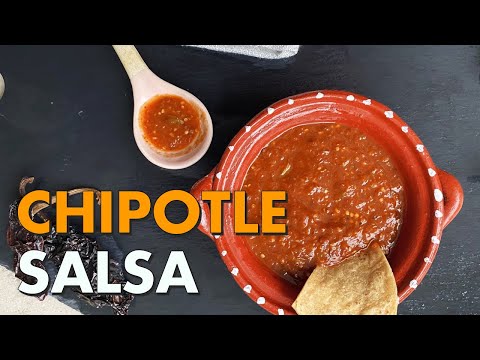The image is a horizontal rectangle with black bars framing the top and bottom. At its center, a realistic photograph features a vibrant depiction of Chipotle salsa text and a bowl of salsa. The background appears to be a black table, adding contrast to the colorful elements. In the bottom left corner, the word "Chipotle" is prominently displayed in bold, orange capital letters, followed by "salsa" in white letters, both bordered in black.

Dominating the right side of the image is a red, sturdy-looking bowl, likely porcelain, adorned with small white dots along its rim. The bowl contains rich, red salsa, with a tortilla chip partially dipped into it from the bottom right. On top of the bowl sits a white spoon, partially filled with the salsa, positioned towards the top left. Subtle scratches and indistinct white objects mar the table's surface, adding texture to the background, while chili peppers seemingly peek out from behind the text, enhancing the image's spicy theme.